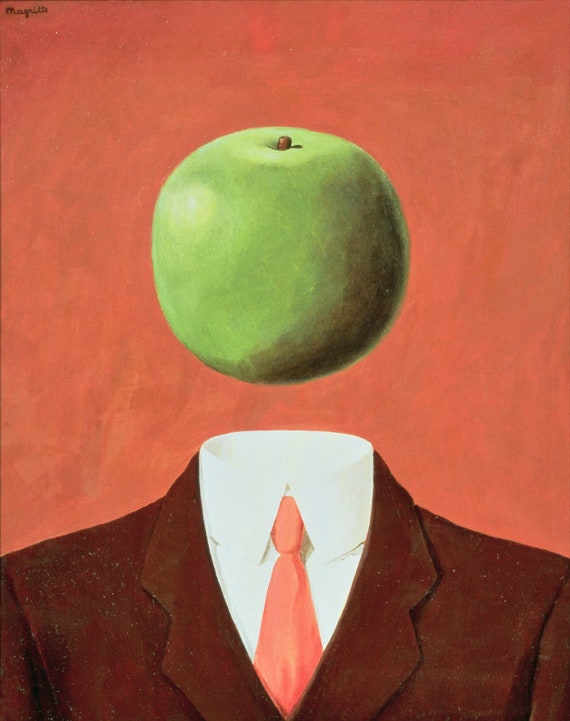This detailed painting, with a red background, portrays a headless figure clad in a dark brown suit paired with a white dress shirt and a neatly tied red necktie. The tie, partially obscured by the suit, has subtle shadows along its edges. Notably, the head is replaced by a floating green apple, embellished with a dark green shadow on the right side and a brown stem. The apple hovers just above the collar of the shirt, suggesting the presence of an invisible neck. The painting, reminiscent of René Magritte's surreal work, appears aged, with signs of wear, and bears the signature "Magritte" at the top.